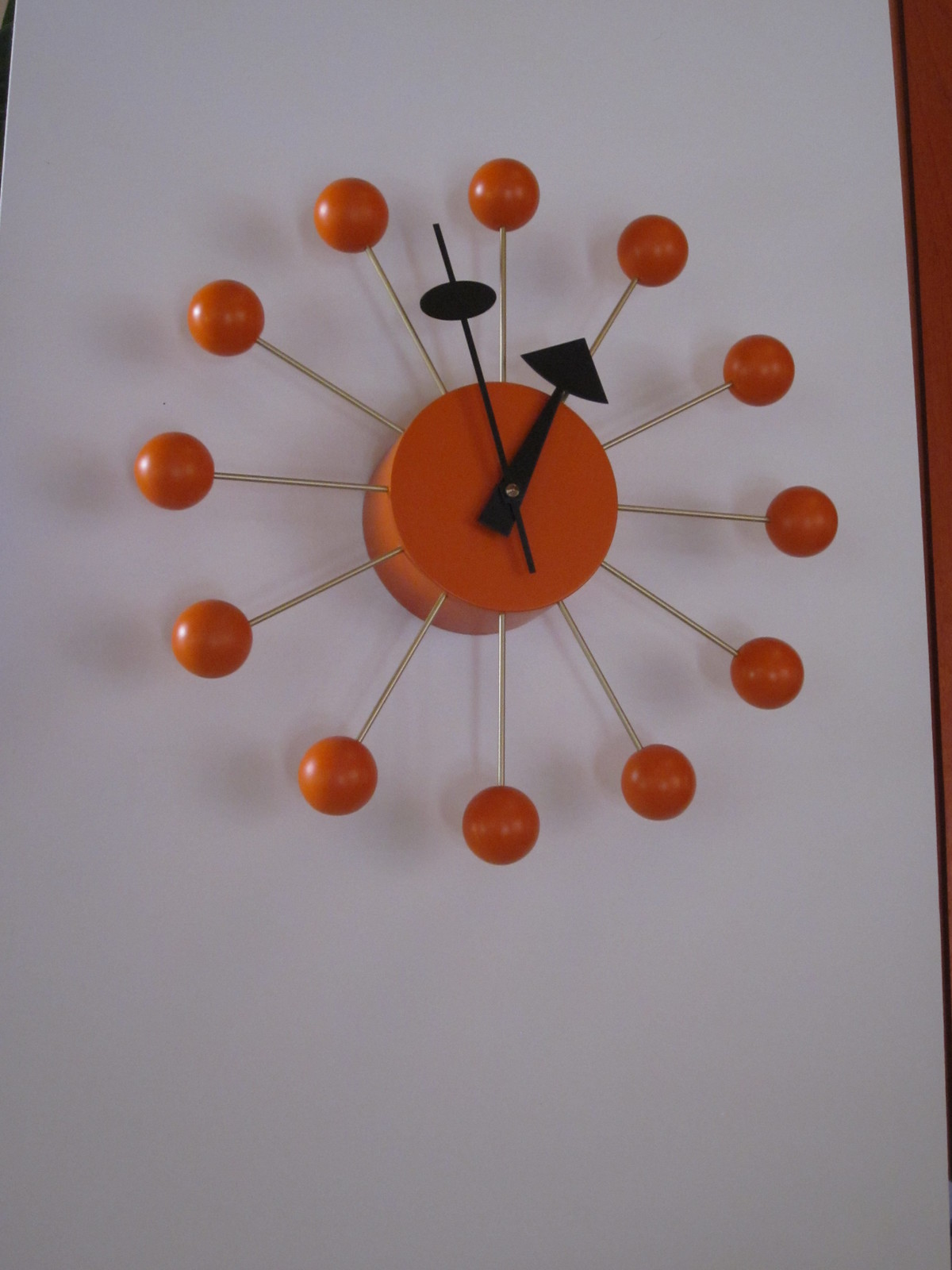A unique and whimsical artistic clock features a circular base from which colorful lollipops extend outward like playful spokes. At the center of the clock, an arrow-shaped hand pivots around a small hole adorned with a black lollipop-like ornament. The time is indicated as one o'clock by the position of the singular arrow hand, adding an extra layer of charm to this imaginative timepiece.